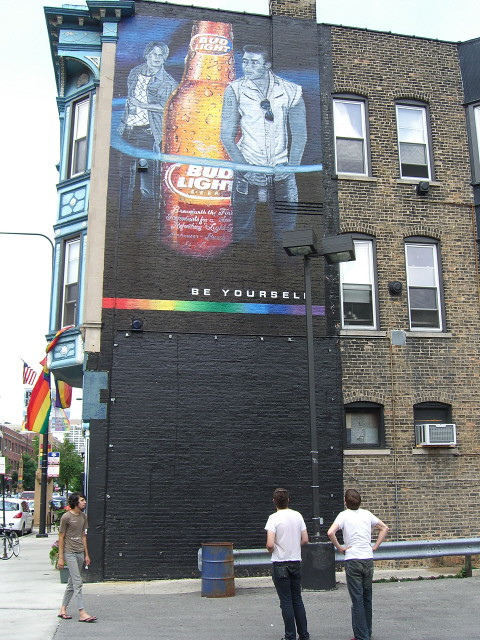In this outdoor photograph taken during the day, we observe a large, brick building primarily in a grayish-brown hue. The structure is divided visually into two distinct sections: the left side features a large, painted black portion with a graphic at the top, while the right side displays four windows and an air conditioning unit. Prominently on the black-painted section is a large, glistening Bud Light bottle, adorned with Bud Light logos on both the neck and label.

Adjacent to the bottle, two men are depicted, appearing smaller in comparison to the oversized bottle image. The man in the back is dressed in a long-sleeved shirt layered over a white shirt, along with pants, while the man in front sports a sleeveless white shirt with a pair of sunglasses hanging from the collar and dark pants. A blue light accentuates their figures, and beneath them, the phrase "Be Yourself" is emblazoned in white letters, accompanied by a horizontal rainbow stripe symbolizing LGBTQ+ pride.

In front of the building, on a sidewalk, three individuals are seen: two of them, with dark brown hair, white shirts, and blue jeans, stand looking up at the graphic. The person closest to the right has a lighter shade of pants and their hands on their hips. A third person, with darker skin, black hair, and a brown shirt paired with grayish pants, walks towards the other two. Additionally, a gay pride flag hangs from the building, and a blue metal garbage can is visible on the sidewalk. Parked cars line the street, and the bright, white sky tops the scene, emphasizing the daytime setting.